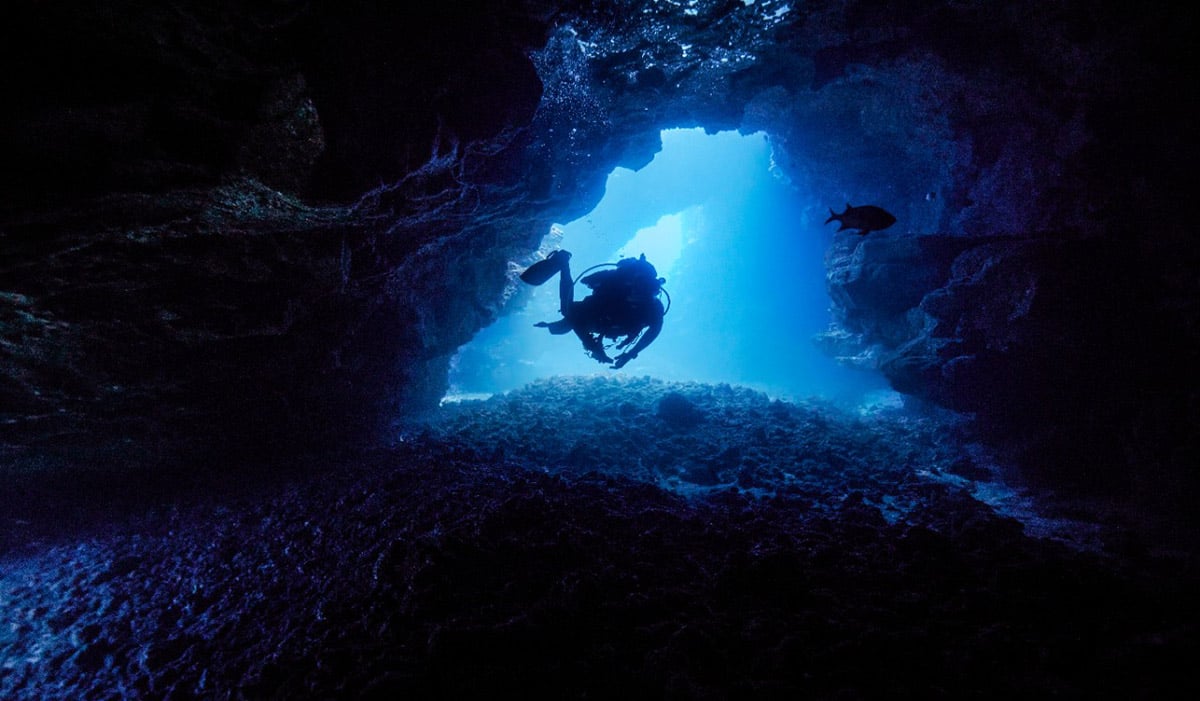In this striking underwater photograph, a scuba diver is captured in silhouette at the center of the image, moving cautiously into an underwater cave. The rocky silhouette of the cave's entrance forms a truncated triangular shape, and the entire image is bathed in a dark blue cast, with the edges considerably darker. The diver, equipped with scuba gear including tanks and hoses visible along with one flipper, is positioned slightly to the left of center, with their hands dangling and feet outstretched, seemingly swimming towards the viewer.

Just to the upper right of the diver, a lone fish floats gracefully, adding a sense of life to the shadowy seascape. The cave's interior is detailed with rocky formations at the bottom, while the area immediately behind the diver is illuminated by a disturbance in the water, enhancing the sense of depth and motion. Despite the overall darkness, the clear lighted water in the middleground highlights the diver and fish, creating a captivating contrast in this serene underwater tableau. It is a dark yet beautiful depiction, encapsulating the mystery and allure of deep-sea exploration.